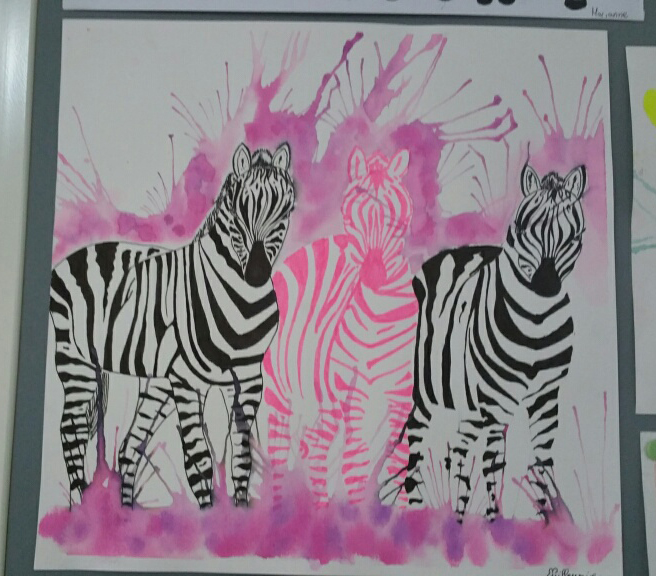The image shows a vibrant watercolor painting hanging on a green wall, likely in a classroom setting. The painting, framed by white trim and partial white pieces of paper at the top and right, depicts three zebras with unique coloration—a central zebra in delicate pink and white flanked by two black and white zebras. They stand on an artistically rendered ground of pink and purple, with similar shades splattered around them in a bushy pattern, creating an expressive backdrop. The zebras, facing forward, exhibit an engaging display, although not anatomically perfect, adding a touch of whimsical charm. The surrounding wall includes hints of additional drawings, indicative of a lively art showcase, possibly from a middle school art exhibition.